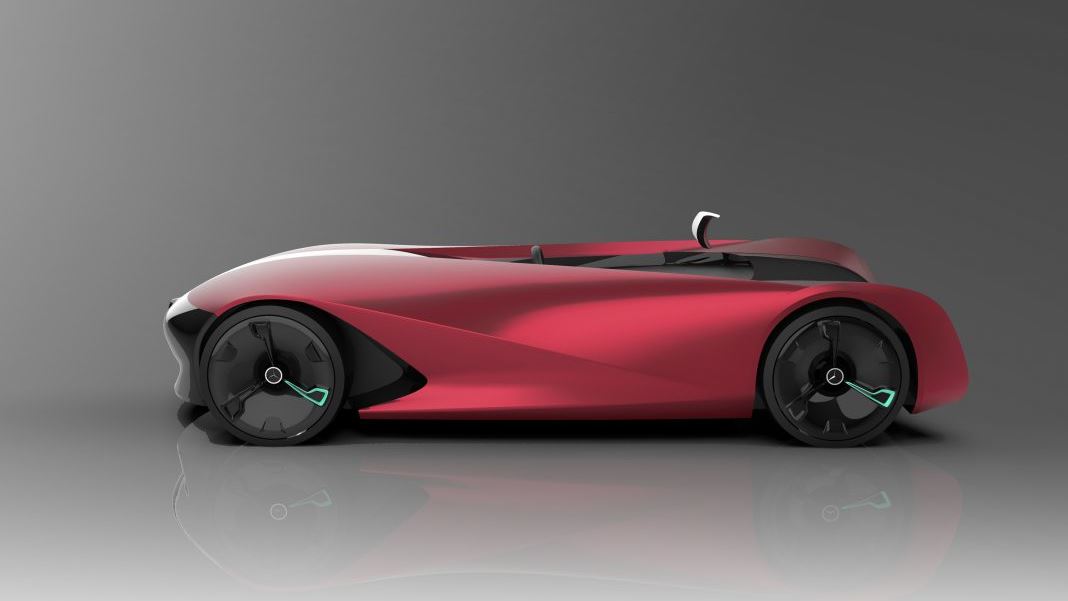The image features a sleek, futuristic vehicle, set against a gradient gray background. The car is striking in its aerodynamic design, appearing both minimalistic and advanced, reminiscent of a futuristic cyber vehicle or a cutting-edge race car. The car's primary color is a vivid red with lighter red accents, contributing to its modern and eye-catching appearance. The black tires are smooth with no visible rims, adding to the vehicle's streamlined look. Notably, the car lacks a roof, suggesting it could be a convertible or an open-top design. The interior is black, with a partially visible black steering wheel and a unique chrome element shaped like a comma emerging from the area where the back seat would be. The vehicle's clean design and detailed features, including a silver fender at the front, make it ambiguous whether it’s a real car or a meticulously crafted toy, giving it an aura of a high-concept advertisement.